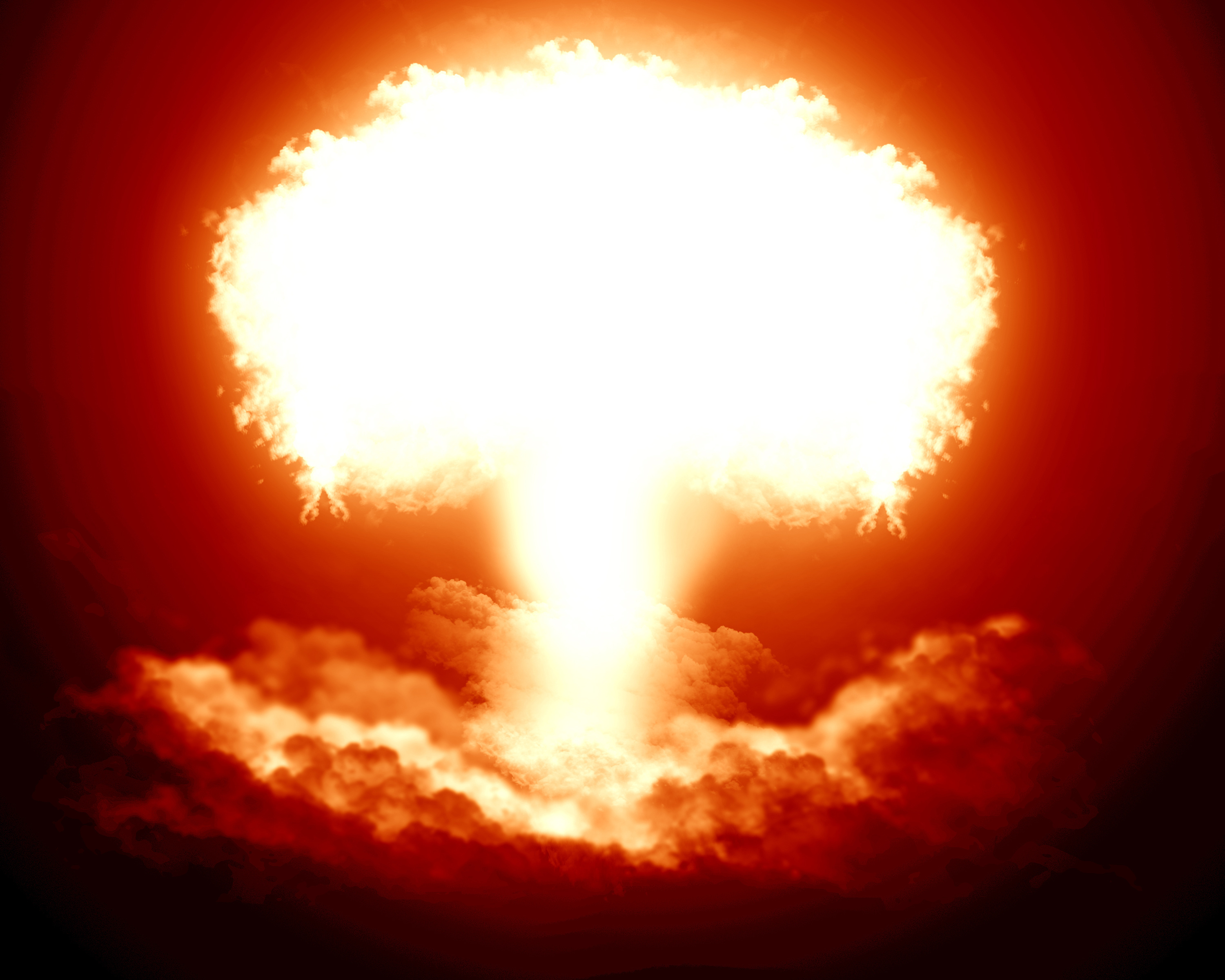The image depicts a photorealistic and possibly edited scene of a nuclear explosion, as characterized by its iconic mushroom cloud. At the center of the frame, the mushroom cloud is vividly portrayed in bright yellow and white hues, which illuminate the entire scene with an intense, almost blinding light. Surrounding the cloud is a gradient radiating outwards, transitioning through shades of orange and dark amber to deep brown and black at the edges.

Beneath the mushroom cloud, plumes of smoke display varied shades of white, orange, and red, contributing to the dramatic intensity of the explosion. The vivid depiction of this fireball-shaped mushroom cloud appears to light up the entire sky, emphasizing the powerful and destructive nature of the event. The image omits any background elements such as human activities or signs of nature, focusing solely on the imposing, central explosion.